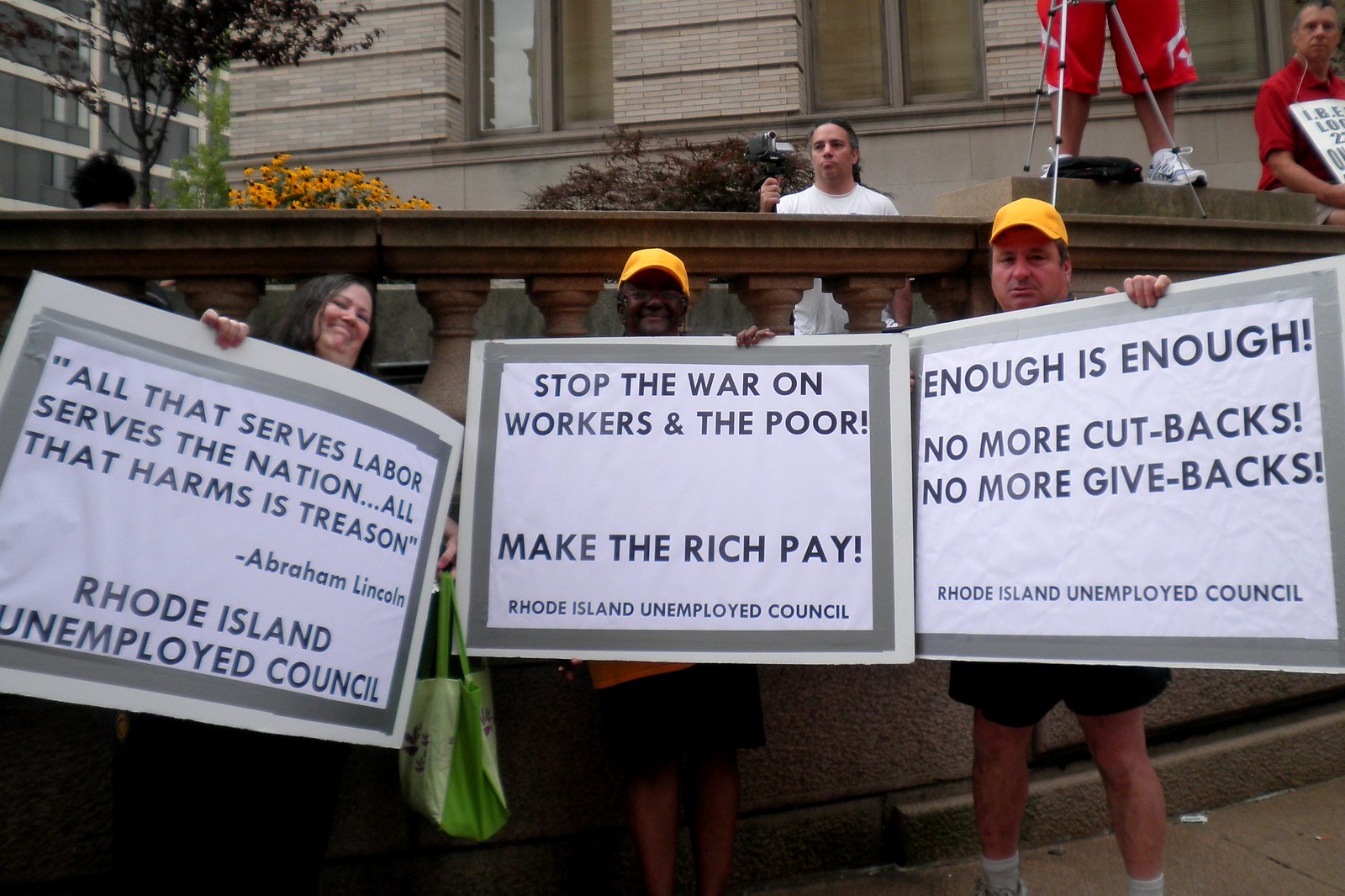In the image, a group of three protesters stands on a sidewalk, holding large signs in front of a building. Each person’s face is visible above their respective sign, which they hold high. The signs are attached with duct tape to pieces of cardboard.

On the left, a woman with a tilted head and a green tote bag holds a sign quoting Abraham Lincoln: “All that serves labor serves the nation. All that harms is treason.” Below this, it states “Rhode Island Unemployed Council.” To her right, a black gentleman in shorts and a yellow ball cap holds a sign that reads, “Stop the war on workers and the poor. Make the rich pay. Rhode Island Unemployed Council.” On the far right, another man, also wearing a yellow ball cap and shorts, holds a sign that says, “Enough is enough. No more cutbacks, no more givebacks. Rhode Island Unemployed Council.”

Behind the protesters is a railing, with people gathered on the other side. Among them are members of the media, including a person with a camcorder and another with a tripod set up. The scene includes elements like yellow flowers visible near the gentleman holding the camera. The overall atmosphere captures the tension and determination of a protest focused on labor rights and economic justice.